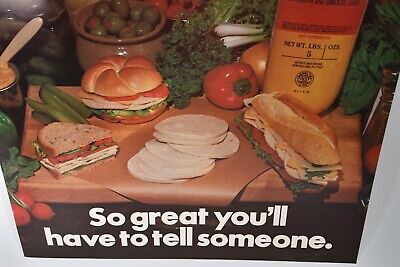The image showcases a deli-style spread arranged on a wooden butcher block table. There are three sandwiches featured prominently: on the left, a half sandwich made with rye bread containing turkey, lettuce, and tomato; in the back left, a round bagel sandwich filled with similar ingredients; and on the right, a small sub sandwich also containing turkey, lettuce, and tomato. In the center of the table, there is a scattered stack of turkey slices. Surrounding the sandwiches are fresh vegetables, including tomatoes, bell peppers, and spinach leaves. Additional items in the background include peppers, pickles, a bowl, a brown jar of olives, and a yellow mustard bottle in the back right corner. The scene is completed with white lettering at the bottom that reads, "So great you'll have to tell someone."